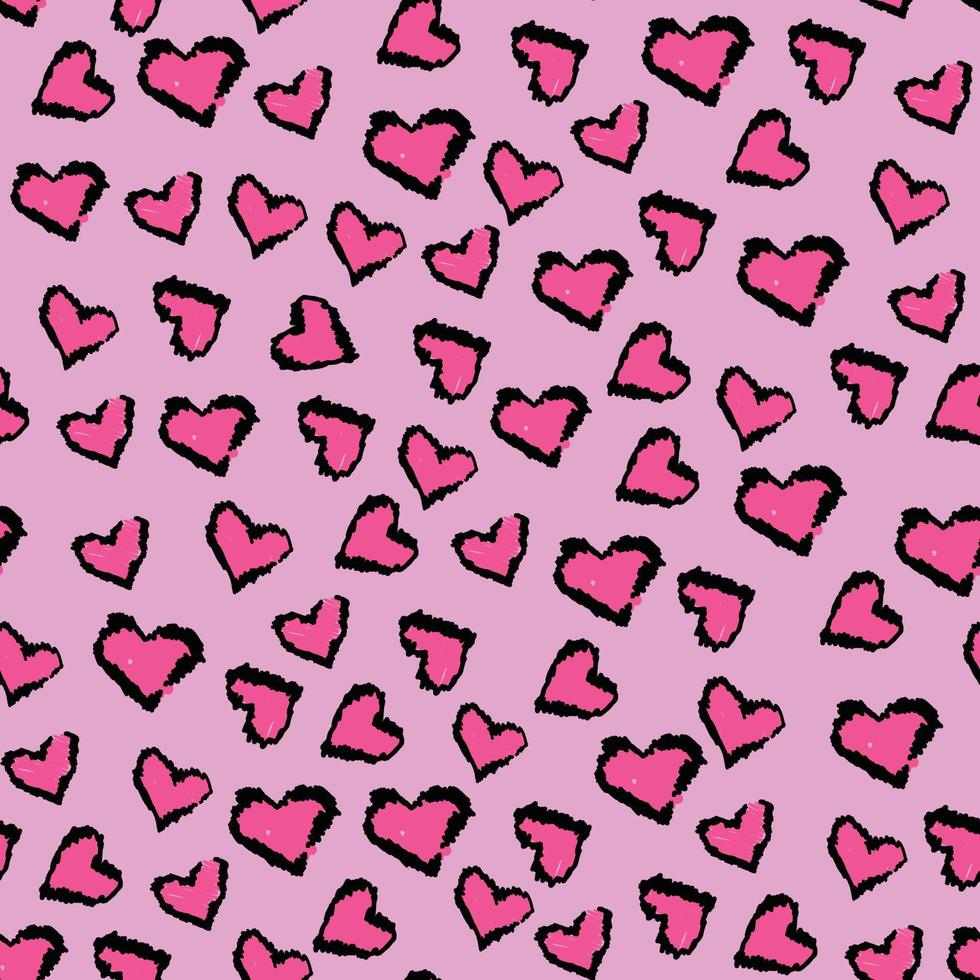This illustration features approximately 50 to 60 dark pink hearts with varying black outlines against a light pink, almost slightly purple, background. The background is uniform in color from top to bottom and left to right. The hearts vary slightly in size, with larger hearts generally having thicker black outlines, while smaller hearts have thinner outlines. The black outlines around the hearts are not uniform; they are thicker in some areas and thinner in others, with occasional breaks and small imperfections in the coloring. Some hearts exhibit little specks or scratches within them. The hearts are oriented in random directions and are densely packed, covering about 50% of the background. The overall arrangement creates an energetic and playful pattern that could resemble leopard print but distinctly uses hearts instead. Edges of some hearts are cut off, suggesting the illustration is framed within a perfect square, hinting that this pattern could exist on fabric, wrapping paper, or as a digital design.